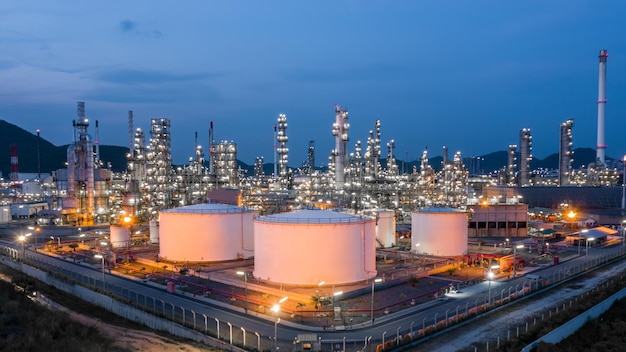The aerial view captures a well-lit industrial facility, likely an oil refinery, nestled against a backdrop of small, darkened mountains or hills. The photograph, taken at a gentle slope just after dusk, reveals a large, square-shaped layout bordered by a road and bound by two layers of high-security fencing reminiscent of a prison. Multiple cylindrical white tanks dominate the foreground, possibly containing crude oil or finished products, with two large tanks flanked by three smaller ones. The background is punctuated by numerous well-illuminated towers and fracking structures. The sky, a dark bluish-gray, contrasts with the extensive lighting throughout the facility, highlighting its intricate apparatus against the twilight.